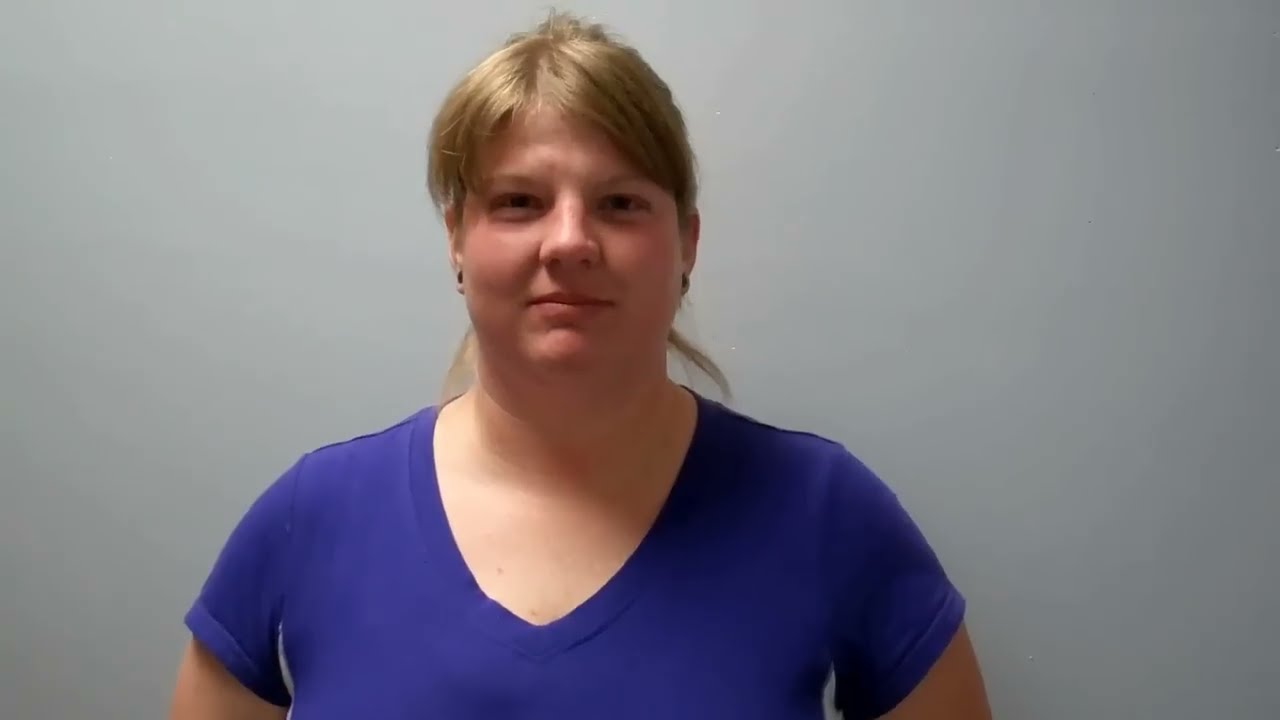The image depicts a young white woman standing slightly left of center against a gray wall that features a subtle gradient effect, brightest right behind her head and darkening outward. Her dirty blonde hair, which is parted slightly off center, is tied into a ponytail. She wears dark earrings and a blue short-sleeved shirt with a deep collar, although there is some ambiguity as others described the shirt as dark purple. The woman has a slight, closed-mouth smile with her eyes slightly narrowed. The photograph captures her from about the bosom upwards, and she appears to be in a neutral setting, perhaps intended for a formal document like a driver's license or passport photo, or possibly as part of a virtual meeting profile.